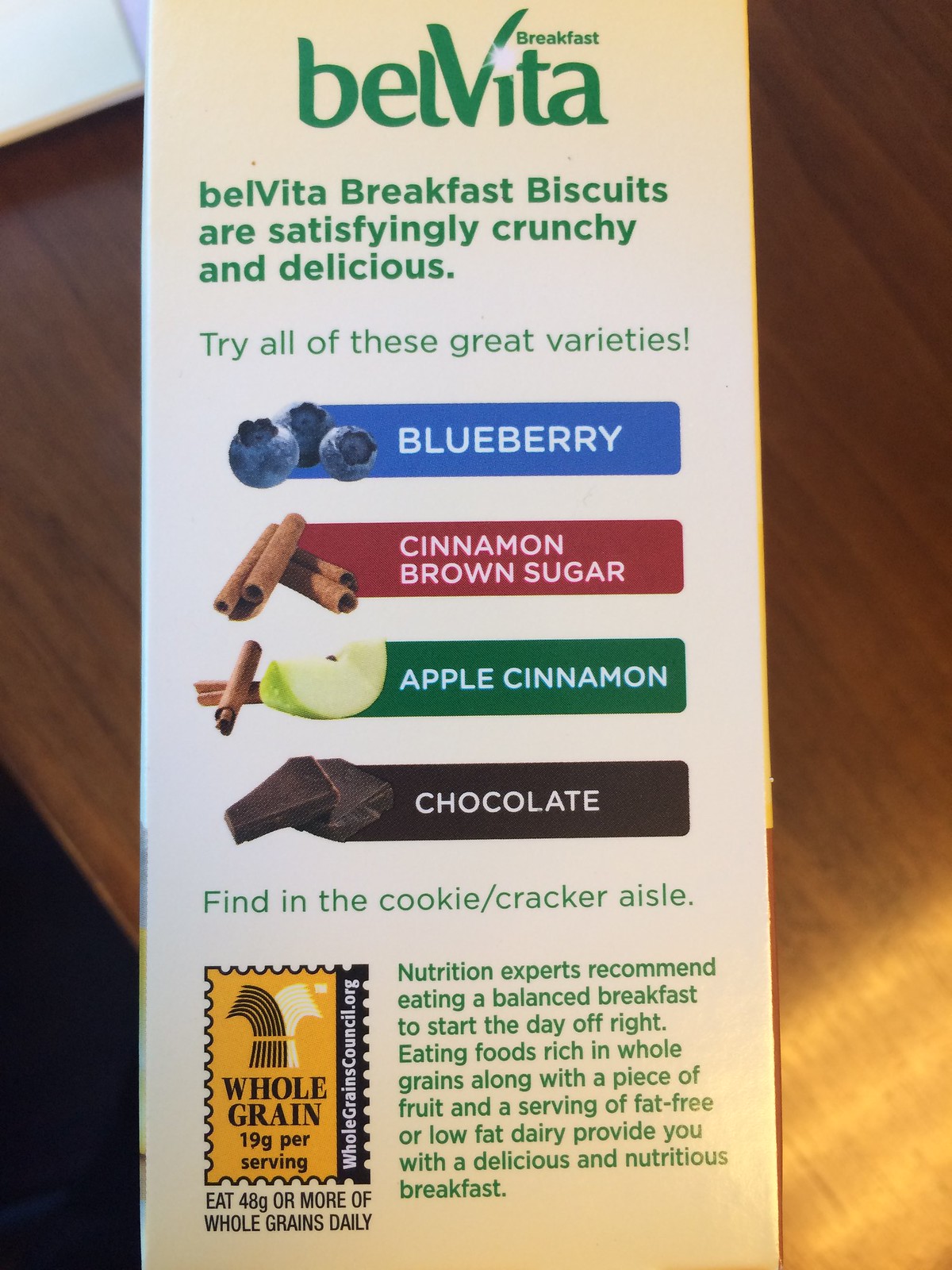The image is a photograph depicting the side of a white paper box of Belvita breakfast biscuits, positioned on a wooden tabletop. The packaging highlights the variety of flavors available: blueberry (illustrated on a blue stripe), cinnamon brown sugar (on an orange stripe), apple cinnamon (on a green stripe), and chocolate (on a dark brown stripe), each accompanied by small images and labeled in white lettering. The text emphasizes that Belvita breakfast biscuits are satisfyingly crunchy and delicious, inviting consumers to try all these great varieties. The box also features a label indicating that the biscuits are made with whole grains. Additionally, it includes a recommendation from nutrition experts about starting the day with a balanced breakfast. It suggests consuming foods rich in whole grains along with a piece of fruit and a serving of fat-free or low-fat dairy for a delicious and nutritious breakfast. It further advises eating 46 grams or more of whole grains daily. The product can be found in the cookie/cracker aisle.